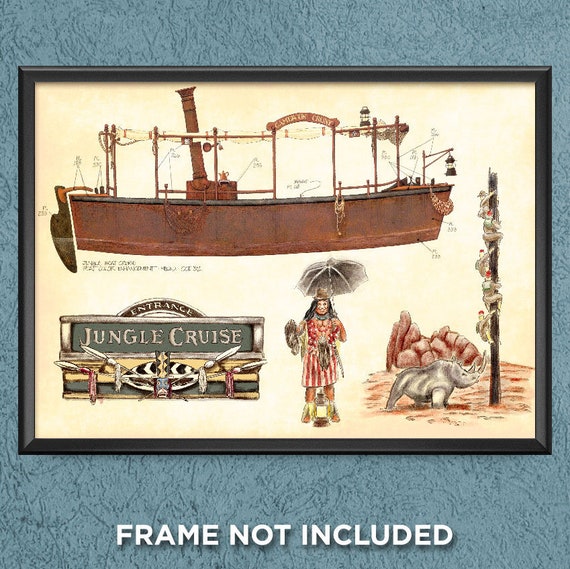This image features a detailed illustration within a black frame, set against a bluish-green stucco-textured wall, with the text "frame not included" at the bottom. The illustration is divided into four distinct scenes, each depicting elements from the Jungle Cruise ride at Disneyland. At the top, an old-time brown boat, resembling an iron fishing vessel, is shown with an engine at the back, a lantern hanging at the front, and various unreadable labels indicating different items on the boat. Beneath this, a wooden sign reads "Jungle Cruise Entrance," adorned with spears and artifacts. In the center, a native figure holds a parasol and is dressed in traditional attire, with a lantern at their feet and possibly a pelt in hand. The bottom right scene portrays a rhinoceros at the base of a tall tree trunk, with five jungle explorers or monkeys in hats frantically climbing to escape, while rocks loom in the background. The entire poster is designed with an aged, yellowed appearance to evoke a vintage feel.